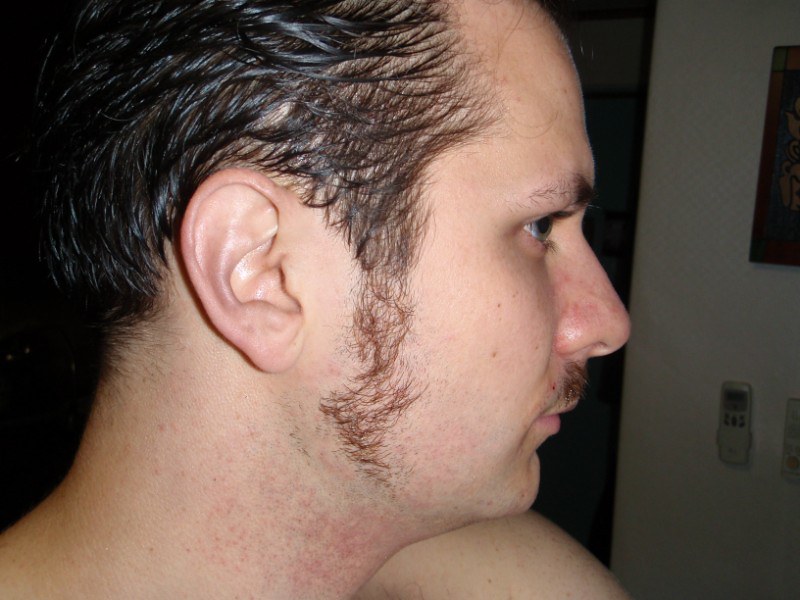The image features a young man, likely in his late 20s or early 30s, with short, dark brown hair. Captured indoors, the photo presents a side profile view of his head, aligned to the left-hand side of the frame, facing towards the three o'clock position. His facial expression is neutral, highlighting his styled facial hair. His beard is creatively trimmed into a triangular shape at the bottom of his sideburns, which extend down to his chin, and he retains most of his mustache. He has bushy eyebrows, prominently dark hair, full cheeks, and a somewhat recessed chin. His bare left shoulder is visible, hinting that he may have just gotten out of the shower or is preparing to get in. Additionally, there are signs of razor burn on his neck. The overall composition of the image is primarily focused on showcasing his detailed facial hair styling.